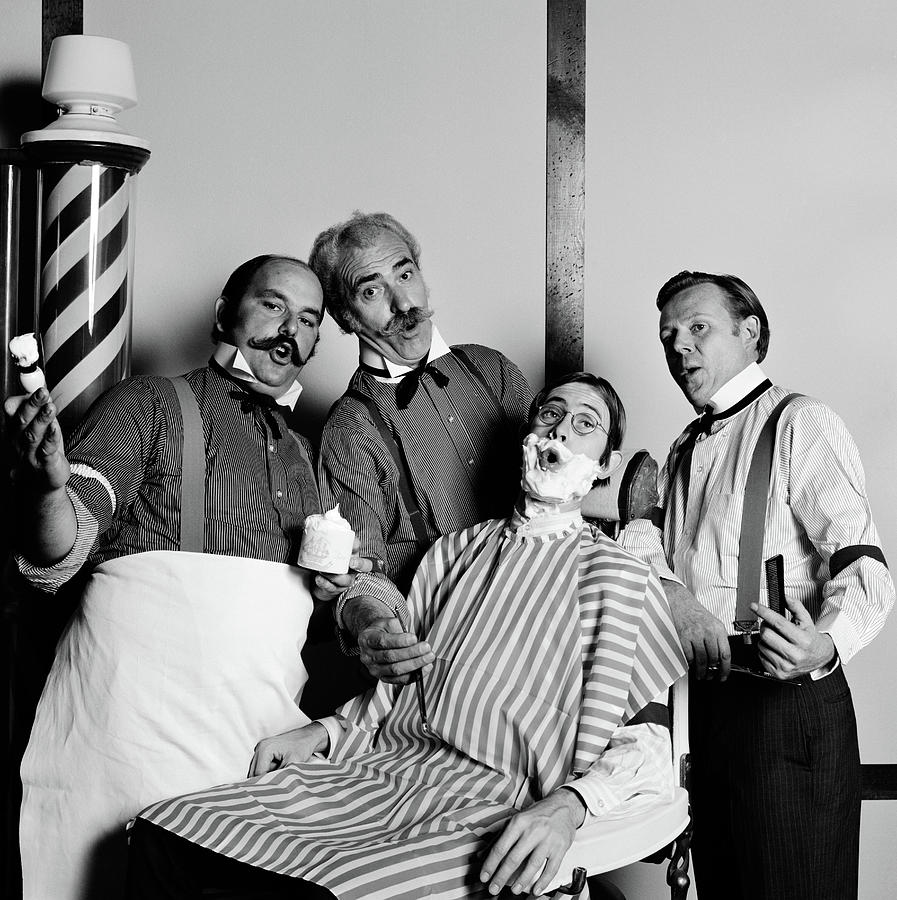The black-and-white photograph captures a lively barbershop quartet scene set in an old-fashioned barbershop. The central focus is a barber, clad in an apron and suspenders, applying shaving cream from a cup to a seated gentleman with a brush. The gentleman has round glasses and a face covered in shaving cream. Surrounding them, three other men, also in suspenders and button-up shirts with bowties, are positioned as if they are singing in harmony. Two of these men sport curly mustaches, while the third is clean-shaven. The men’s collars are stylishly fastened high up their necks, adding to the vintage feel. A traditional barber pole on the left side of the image, with its signature red and white stripes, spins to indicate the classic barbershop setting. All the subjects have open mouths, engrossed in singing, epitomizing a barbershop quartet performance.